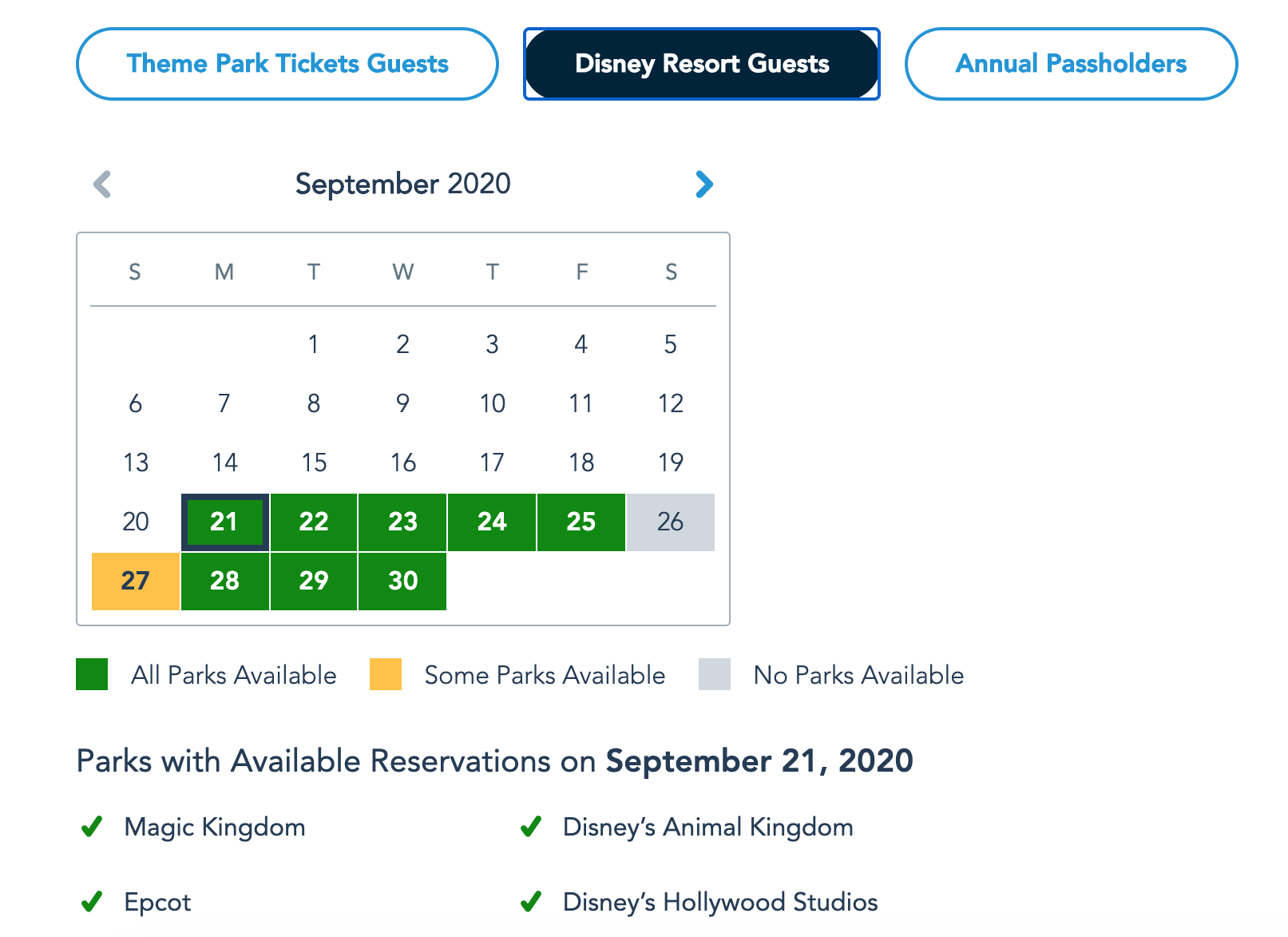This screenshot features a user interface with a white background. At the top, there are three horizontal, oval-shaped buttons outlined in blue with blue text. From left to right, these buttons read: "Theme Park Tickets Guest," "Disney Resort Guest" (which is selected, indicated by a black background and white text), and "Annual Pass Holders."

Approximately five lines below, a gray left-pointing arrow is seen. Below this arrow is a calendar with the text "September 2020" in bold black, centered above the calendar. On the right side of the calendar header, there is a blue right-pointing arrow. The days of the week, abbreviated as SMTWTFS, are listed at the top of the calendar grid, beginning with Sunday.

The calendar starts on Tuesday, the 1st, and displays the entire month up to the 30th. Specific dates — the 21st, 22nd, 23rd, 24th, 25th, 28th, 29th, and 30th — are highlighted with green squares, containing white numbers. Additionally, the 26th is marked in gray, and the 27th is highlighted in yellow.

Below the calendar, there is a color-coded key: a green square followed by the text "all parks available" in gray, a yellow square followed by "some parks available" in gray, and a gray square followed by "no parks available" in gray.

Approximately three lines below the key, the text "Parks with available reservations on" is in black, followed by a bolded "September 21, 2020." Beneath this, a list of parks with green check marks indicating availability includes:

- Magic Kingdom (green check, left)
- Disney's Animal Kingdom (green check, right)
- Epcot (green check, four lines down)
- Disney's Hollywood Studios (green check, right)